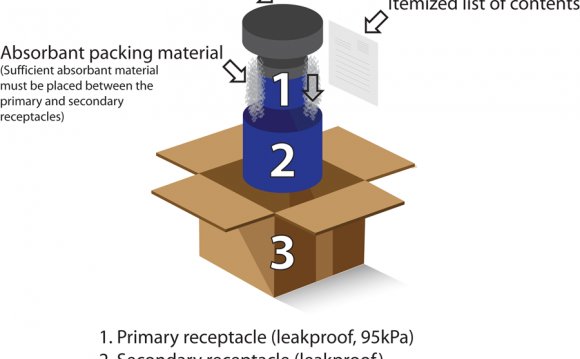This detailed 3D illustration on a white background depicts an open brown cardboard box with a blue and gray cylindrical object hovering above it, appearing to be placed into the box. The image is annotated with various arrows and numbered indicators. The cylinder has three numbers: '1' at the top, '2' at its base, and '3' in front of the open box. The top-right corner features an arrow labeled "Itemized List of Contents" pointing to an illustrated piece of paper. Another arrow on the left side points to the middle of the cylindrical object, labeled "Absorbent Packaging Material," with a note that sufficient absorbent material must be placed between the primary and secondary receptacles. A third arrow on the right side of the cylinder points downward. At the image’s base, the text reads "One Primary Receptacle, Leak Proof 95 KPA," followed by additional, partially cut-off text mentioning the secondary receptacle. The detailed labeling suggests the diagram is instructional, likely showing the correct method for packaging a leak-proof cylindrical item with specified absorbent material for secure transportation.